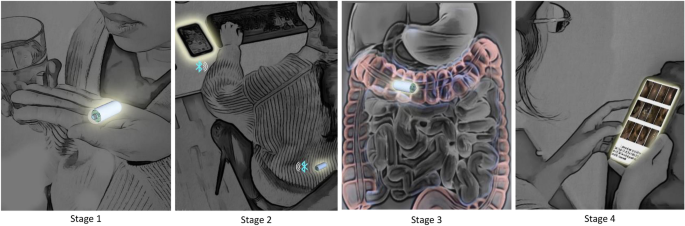The image series comprises four panels labeled Stage 1 through Stage 4, illustrating the journey of a cylindrical medical device through a person's body. In Stage 1, the close-up drawing depicts a woman's black-and-white hand holding a small white cylinder with a green dot, resembling a compact battery. A glass of water is noticeable nearby. In Stage 2, the woman is seated at a desk with a computer and smartphone, showing a Bluetooth icon highlighted on both. The white-and-green cylinder depicting connectivity has seemingly moved inside her body, illustrated by a glowing Bluetooth insignia on her back. Stage 3 transitions to an internal view of the woman's body, specifically focusing on the cylinder traveling through pink, brown, and gray sections of her intestines. Finally, Stage 4 shows the woman examining her smartphone, monitoring the device's progress through a specialized app. This sequence likely represents the swallowing of a medical device, which is then tracked as it navigates through her gastrointestinal tract.